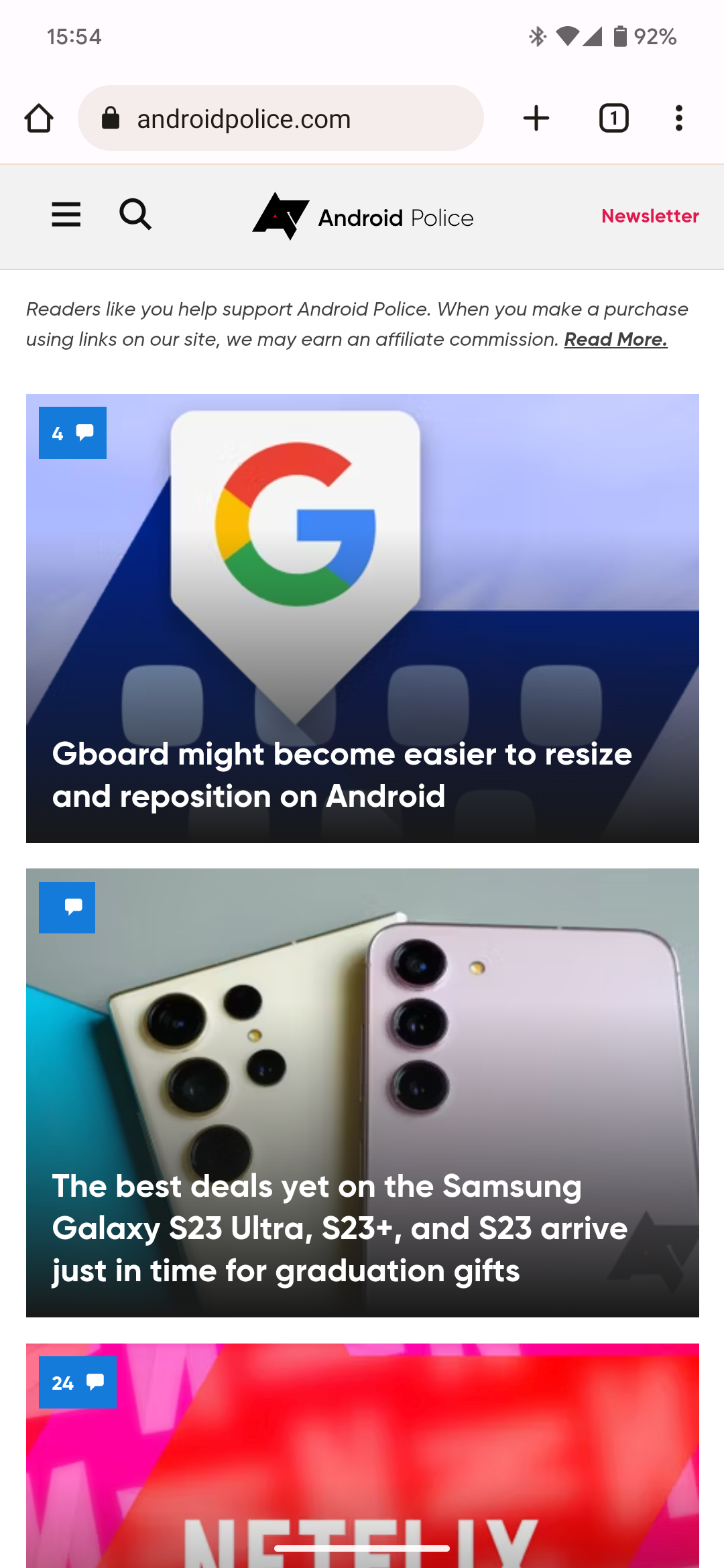This is a screenshot from a smartphone captured at 15:54, showcasing various elements on the screen. To the right, there are icons indicating an internet connection and a battery charge of 92%. Below these icons, a small home button icon is visible. 

The search bar displays a lock symbol on the left, followed by "androidpolice.com." To the right of the URL is a plus sign (+), a square with the number one inside, and three vertical dots for more options. 

Underneath the search bar, there is a gray navigation bar with three horizontal lines on the left, a search icon next to it, and a black symbol representing Android Police. "Android" is written in black, and "Police" is in medium gray. Next to this, there is a red label that reads "Newsletter."

Below this, text states, "Readers like you support Android Police. When you make a purchase using links on our site, we may earn an affiliate commission." This is followed by "Read More" in bold, underlined text.

Following this information, three images are partially visible. The first image has a blue background with a darker blue shape resembling a keyboard and a Google 'G' tag. In the upper left corner, a small blue box with the number four and a comment symbol is present. The caption under the 'G' reads, "Gboard might become easier to resize and reposition on Android."

The second image features two cell phones. The view shows their camera modules, with one phone having three cameras aligned vertically and the other phone featuring the same three vertically aligned cameras, as well as two more cameras to the right and a smaller one in between. The accompanying text reads, "The best deals yet on the Samsung Galaxy S23 Ultra, S23, S23 Plus, and S23 arrived just in time for graduation gifts."

The third image has a red and pink colorful background, but its caption is not fully visible, making it unclear what the image depicts.